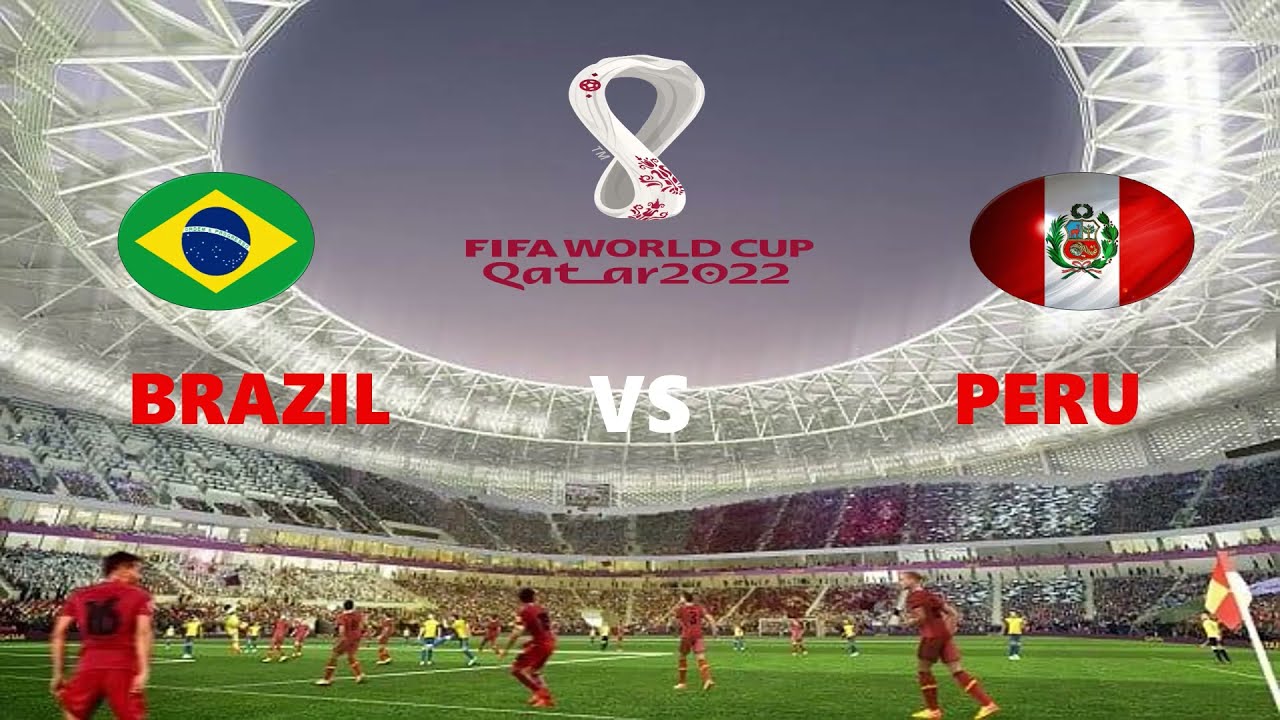The image depicts a lively scene at an outdoor stadium under an open dome, showcasing a professional soccer match between Brazil and Peru. The rich green grass of the field is prominently visible, marked by white lines and goals. The stadium is filled with a vibrant crowd, more densely packed in the lower levels, watching the teams in their respective uniforms—Brazil in dark red and yellow attire and Peru in yellow shirts with blue pants. At the top center of the image, against a purplish sky backdrop, is the official FIFA World Cup Qatar 2022 logo, featuring a distinctive upside-down white infinity symbol adorned with a red floral pattern. To the left of the logo, the Brazilian flag is displayed in an oval with the text "Brazil" in red letters beneath it. To the right, the Peruvian flag is similarly presented in an oval with the text "Peru" in red letters beneath it. Between these ovals, the word "versus" is prominently shown in white letters, emphasizing the competitive encounter.